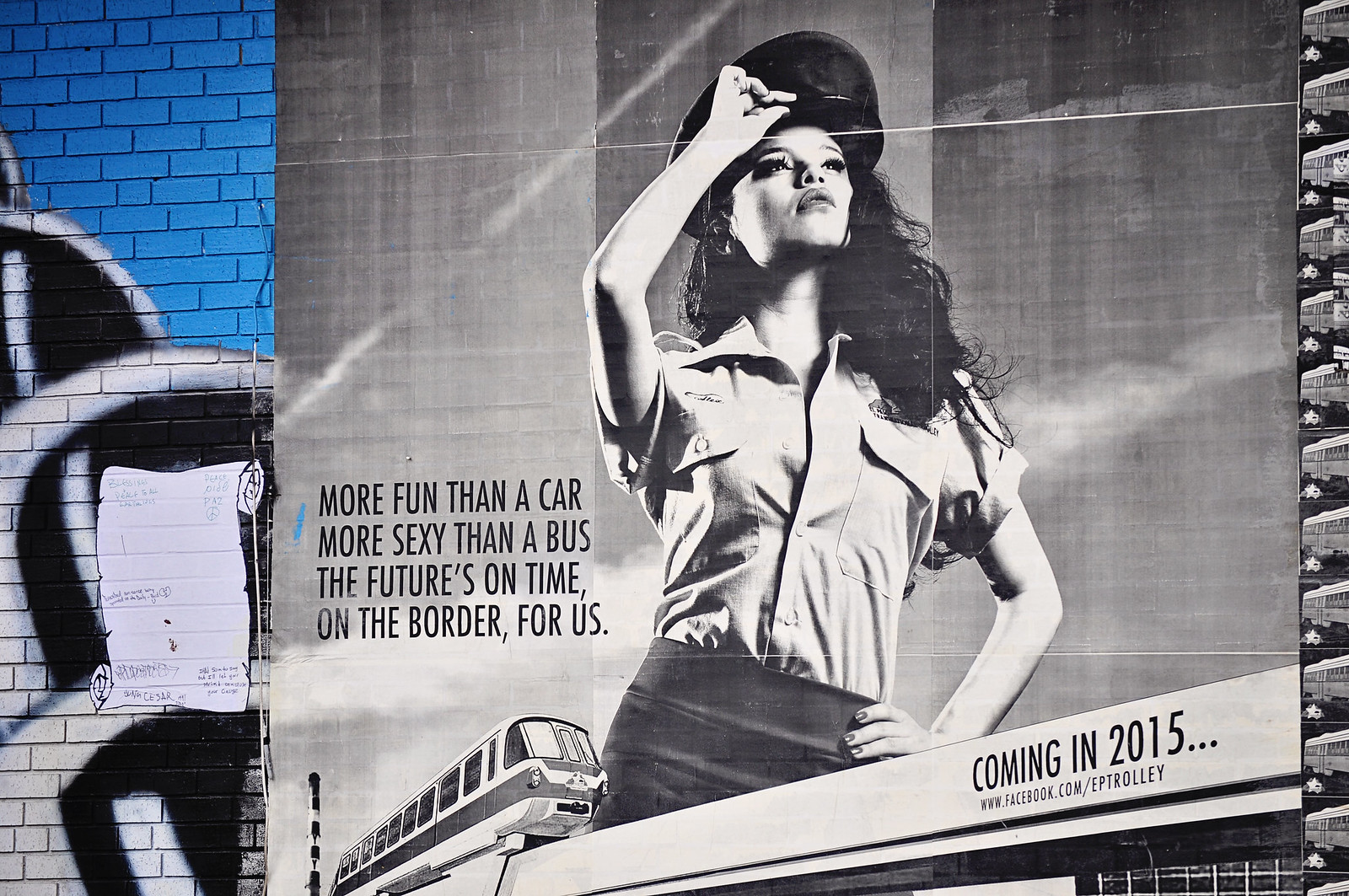The image showcases a promotional advertisement painted on the side of a blue brick wall adorned with graffiti art. The graffiti features a black and white design, reminiscent of rolled parchment paper. Adjacent to the graffiti are several posters, partially obscuring the brick background. The posters depict a stylish woman wearing a black hat, with long black hair, a button-up shirt, and a skirt. Additionally, a sleek train or trolley, depicted on a high-speed track, is part of the visual. The left side of the advertisement features the text: "More fun than a car, more sexy than a bus, the future is on time for us. Coming in 2015. www.facebook.com/EPTrolley."